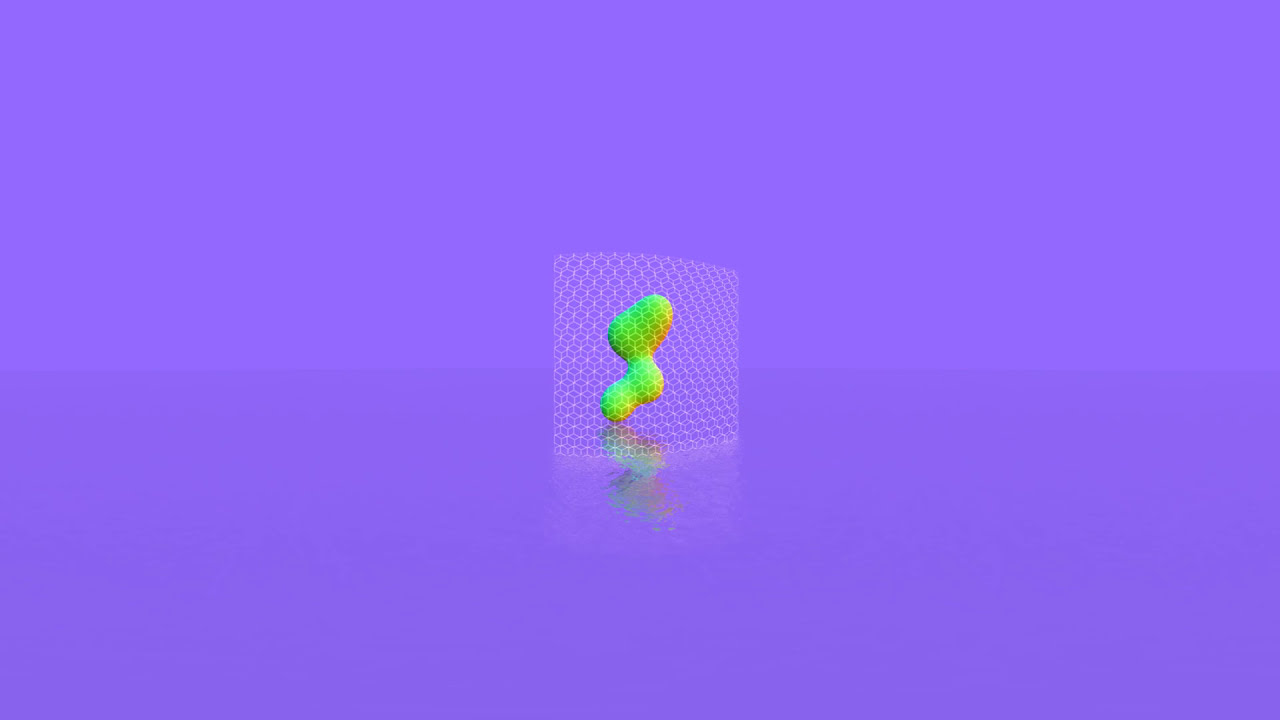The image features a divided blue-to-purple gradient background, with the top half in a slightly lighter hue and the bottom half in a darker tone. At the center of the image is a pixelated, see-through box with an intricate geometric design reminiscent of tessellating patterns or fencing. Inside this box is an iridescent green blob, faintly tinged with yellow and orange at the edges. The blob is ambiguous in shape, resembling a dog bone, a foot, or a chicken leg. The entire scene has a surreal, computer-generated appearance. Beneath the central figure, there's a faint, shimmering reflection, giving the impression of a water texture with subtle ripples. The image overall is very detailed yet abstract, creating a trippy visual effect.